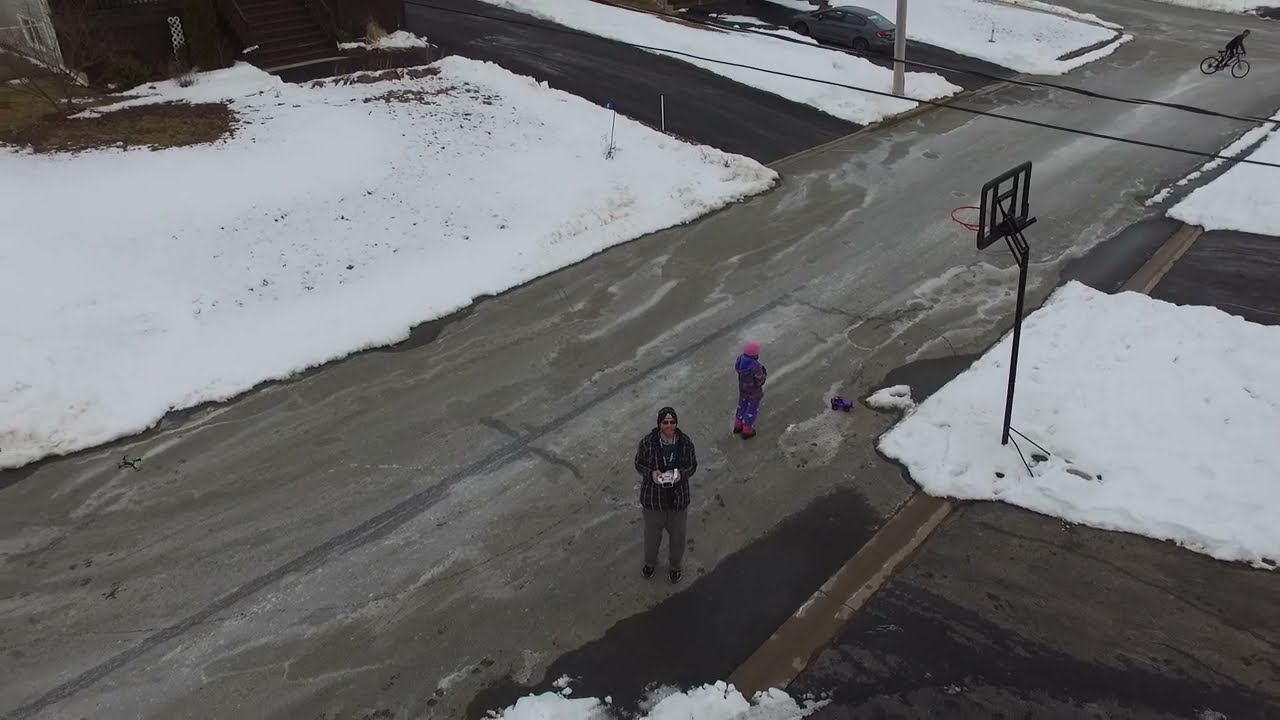The photograph captures an aerial, slightly elevated view of a quaint neighborhood during winter, shrouded in a blanket of snow. The scene unfolds beneath a cloudy, grayish-blue sky, adding to the serene atmosphere. The focal point is a cul-de-sac, with the main road curving from the bottom right corner up towards the top left, where it rounds into a circle. The roads are clear, contrasting with the snow-covered yards and roofs of the houses. 

Flanking the road, there are roughly 10 to 15 unique single-family homes, each varying in size, design, and color. The exteriors range from beige, gray, to red, and their roofs span a palette of red, dark brown, black, and gray. Additional houses encircle the roundabout area at the cul-de-sac's end, maintaining the neighborhood’s eclectic aesthetic.

Scattered throughout the yards and lining the streets are barren trees, adding character to the wintery scene. In one particular yard, an above-ground pool is partially visible, hinting at warmer days. The landscape continues beyond the homes, opening up to more snow-covered land and a backdrop of more trees, leaving a peaceful and picturesque impression.